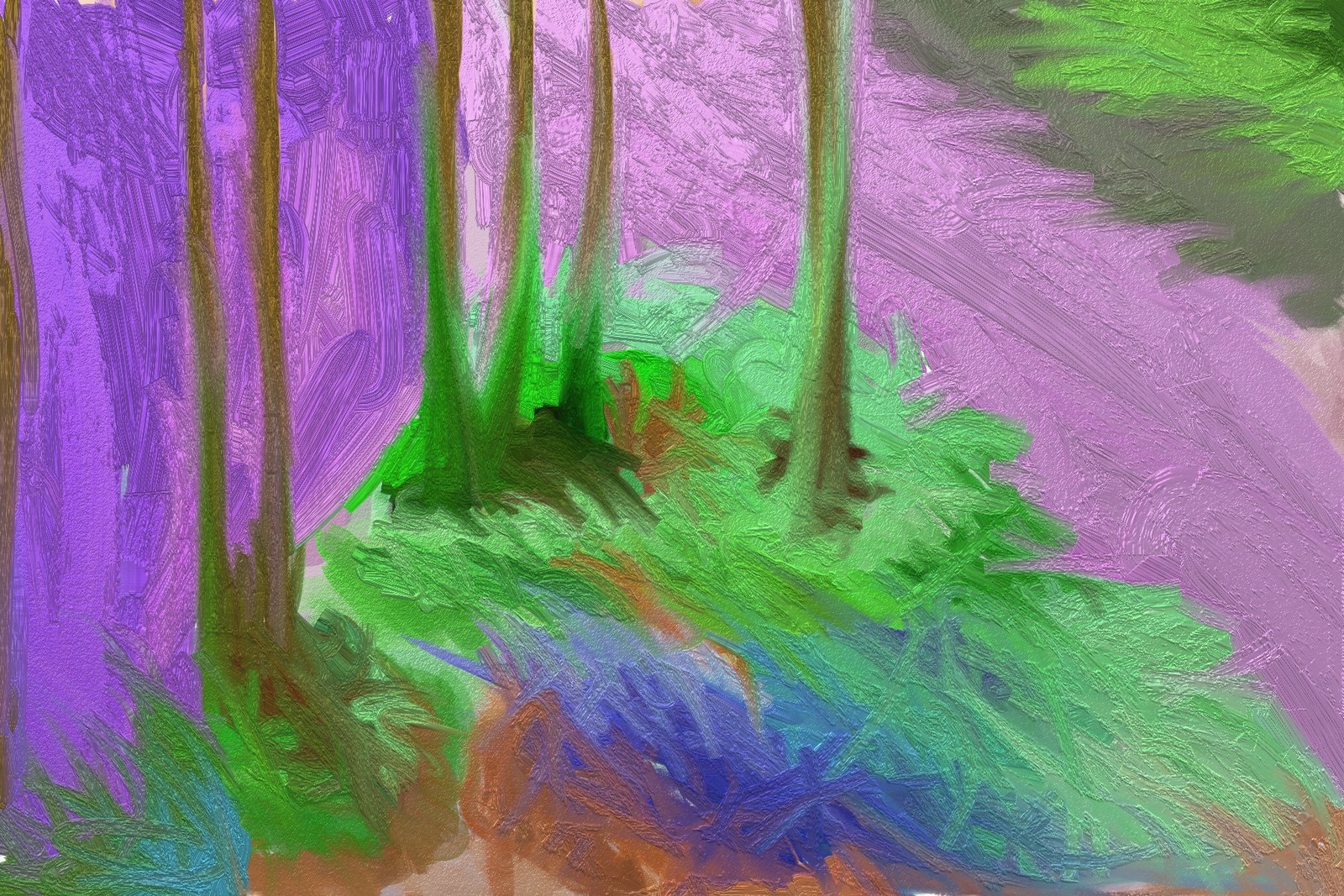This abstract painting features a vibrant and colorful scene that closely resembles an abstract forest. The canvas is filled with a variety of colors, including shades of pink, purple, brown, green, orange, blue, and light blue. The brush strokes are clearly visible, adding a textured dimension as they move in all directions. 

At the center and left side of the painting, there are noticeable abstract representations of tree trunks. Some trunks appear brown and thicker at the bottom, suggesting the sturdiness of a tree base, while others start green at the bottom and transition to brown toward the top. Notably, there are two brown tree trunks standing close together in a cluster of vegetation, three similarly clustered trunks at the center of the painting, and a lone trunk within its own patch of greenery. The overall composition of these trunks forms a unique pattern that is both chaotic and harmonious.

In addition to the tree elements, the painting features green vegetation and blocks of purple hues, alongside green and brown zones that could be interpreted as grass or field sections. A flowing shape resembling a river, painted in purple, starts from the bottom right and moves diagonally to the middle top, delineating a passage through this abstract landscape. Complementing this, the top right section of the painting shows greener hues that contrast with the more muted pastels, enriching this whimsical scene.

Overall, the abstract forest is realized through a mixture of colors and textured strokes, with an interesting interplay between natural elements and abstract forms, possibly created using pastel chalk or a finger-painting technique.